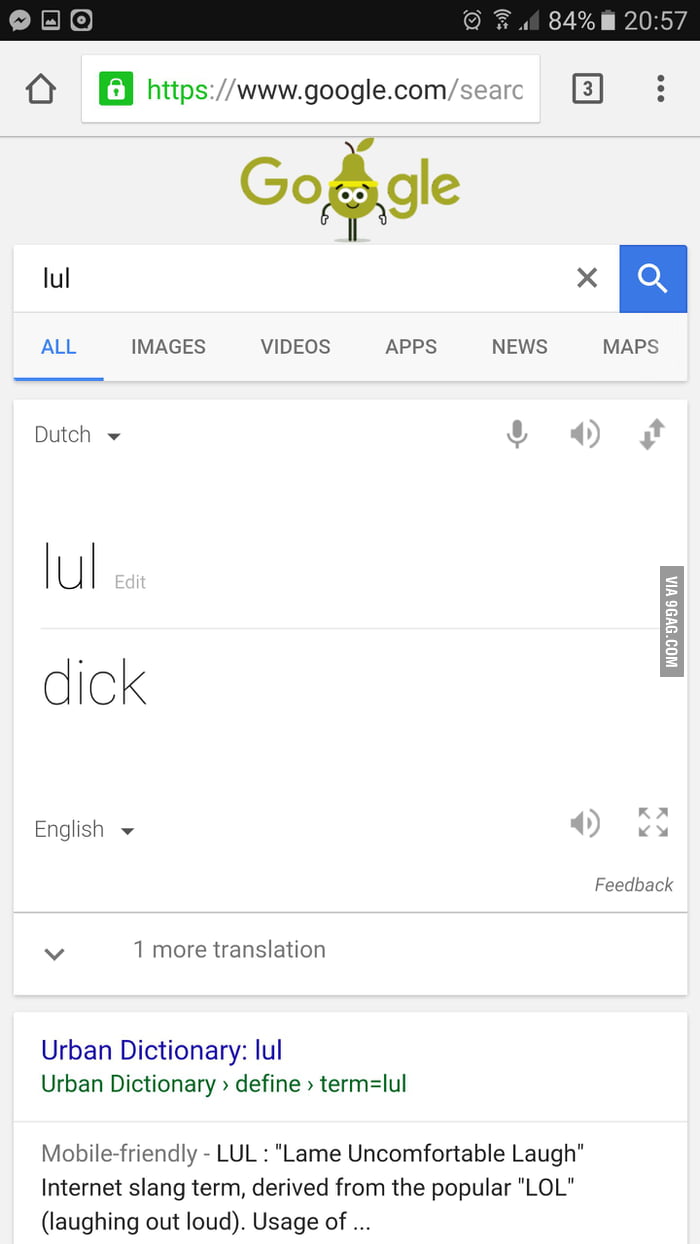Here's a cleaned-up and detailed caption for the image:

---

The image depicts a smartphone screen displaying a web browser currently on the Google search page. 

1. **Top Bar**:
   - **Left Corner**: A black box icon is visible.
   - **Text**: Various items in a gray font are listed on the left.
   - **Right Corner**: Wi-Fi signal strength indicator shows low, an 84% battery icon, and the current time (20:57) all in gray font.

2. **Address Bar**:
   - **Left**: A house icon on the far left.
   - **Right**: Three vertical dots followed by a square with the number three beside it.
   - **Center**: A green padlock icon indicating a secure connection, followed by `https://` in green. The URL `www.google.com/search` is in black text.

3. **Search Section**:
   - **Logo**: The Google logo with a leaf and stem atop the second "O," which has been transformed into a character with black eyes, arms, eyebrows, thin legs, and black outlines.
   - **Search Bar**: Contains the text "LUL" in black font on a white background, followed by a black "X" and a blue search button with the search icon in white.

4. **Navigation Tabs**:
   - **Options**: "All" (highlighted in blue with a blue line underneath), followed by gray tabs: Images, Videos, Apps, News, and Maps.

5. **Language and Tools**:
   - **Left**: The word "Dutch" with a downward-pointing arrow, followed by a gray microphone and speaker icon, and up and down arrows.
   - **Search Result**: The term "LUL" with an "edit" option followed by a gray line. On the right, a gray box with the website `via9gag.com` in white font.
   - **Additional Menu**: On the left, options such as "Dick," "English" (with downward arrow), a speaker icon, and a square with four arrows pointing in different directions.

6. **Bottom Section**:
   - **Feedback and Translation**: "Feedback" with a gray line and a downward-pointing gray arrow on the left. The text "More translations" appears with a gray spacer.
   - **Search Result Description**: The term "Urban Dictionary" followed by green arrows labeled "Define" and "term=LUL." Below that, a gray text reads `Mobile-friendly LUL 'lame, uncomfortable laugh'`, and further explanation states it is an internet slang term derived from "LOL" (laughing out loud).

---

This descriptive caption provides a thorough and organized breakdown of the elements visible on the smartphone screen.